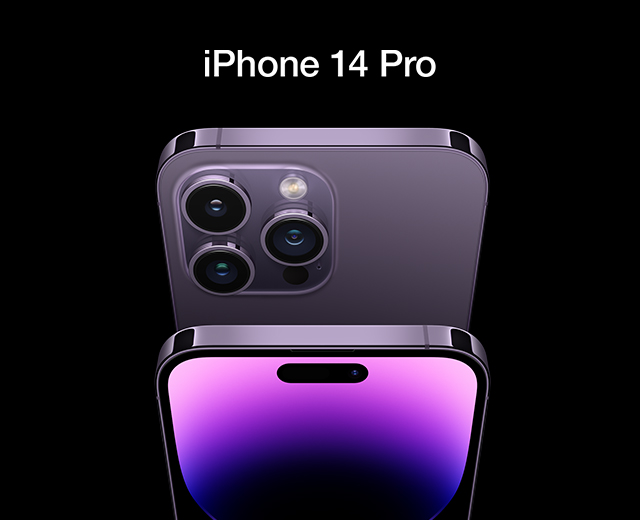This image features an advertisement for the iPhone 14 Pro, set against a sleek black backdrop. At the top center, prominent large white text reads "iPhone 14 Pro." The visual highlights both the top rear and top front of the phone, showcasing what appears to be a silver or purplish-silver model. The back of the phone displays the distinctive camera cluster with two lenses positioned on the top left and a third lens offset to the right, accompanied by the flash above it. Beneath the device, the front screen features a stunning purple gradient transitioning from light to dark, accentuating the phone’s glossy metallic finish. The overall presentation exudes modern elegance and advanced technology.